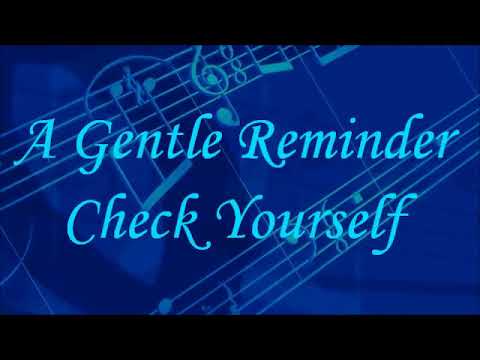The image features a blue rectangle with floating staves and various musical notes set against a black background. The blue rectangle stretches horizontally across the image, leaving visible margins of black on the top and bottom, creating a wide-format screen effect. The staves and notes, depicted in light blue and giving a scrolling, vertical wrap-around appearance, add a dynamic musical element to the background. Overlaying this musical backdrop is a two-line, light blue, scripted-text message. The top line reads "A Gentle Reminder," with each word's initial capitalized, and the bottom line states "Check Yourself," also with initial capital letters. The text style is ornate, with elegant curls and curves adding to its sophisticated look.